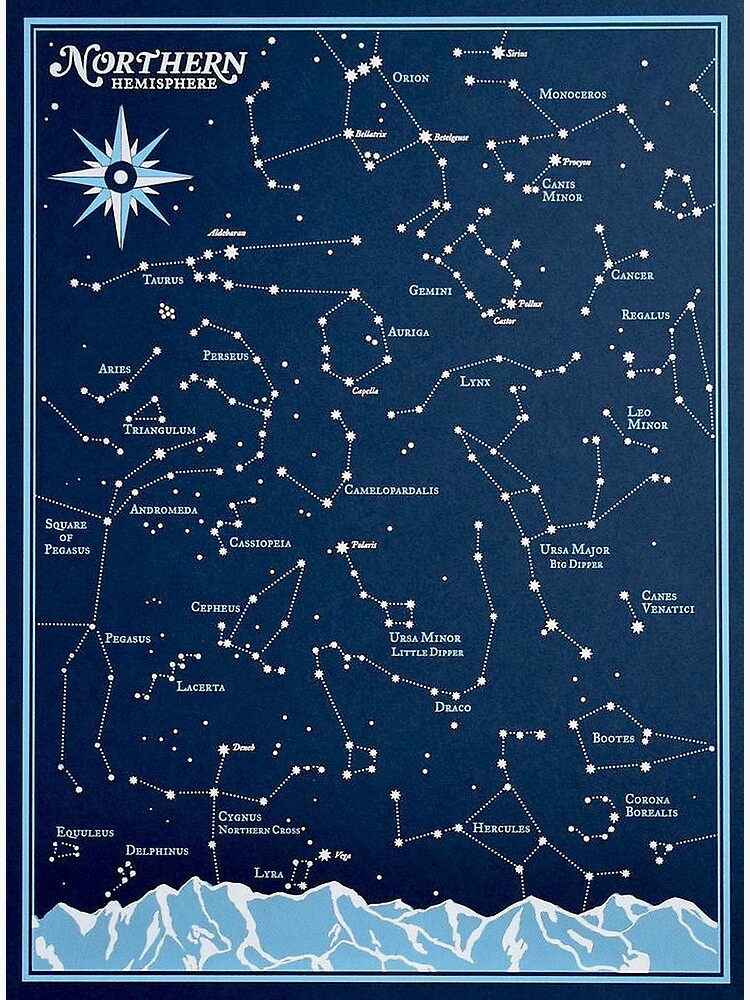The image is a detailed poster depicting the star constellations of the Northern Hemisphere. At the top left corner, the text "Northern Hemisphere" is prominently displayed next to a blue and white constellation-like logo. The background of the poster is a deep, dark blue, accentuating the starry sky, with each constellation meticulously illustrated with white lines connecting the stars. Among the visible constellations are Aries, Leo, Pegasus, Hercules, Ursa Major, Ursa Minor, Cassiopeia, Gemini, and Cancer, among others.

In addition to the intricate star patterns, the lower edge of the poster features a stylized mountain range in light blue and white, resembling snow-capped peaks. This artistic element adds depth to the celestial theme of the poster. Overall, the detailed constellations are labeled clearly against the dark blue backdrop, making it both a visually captivating and informative guide to the Northern Hemisphere's night sky.